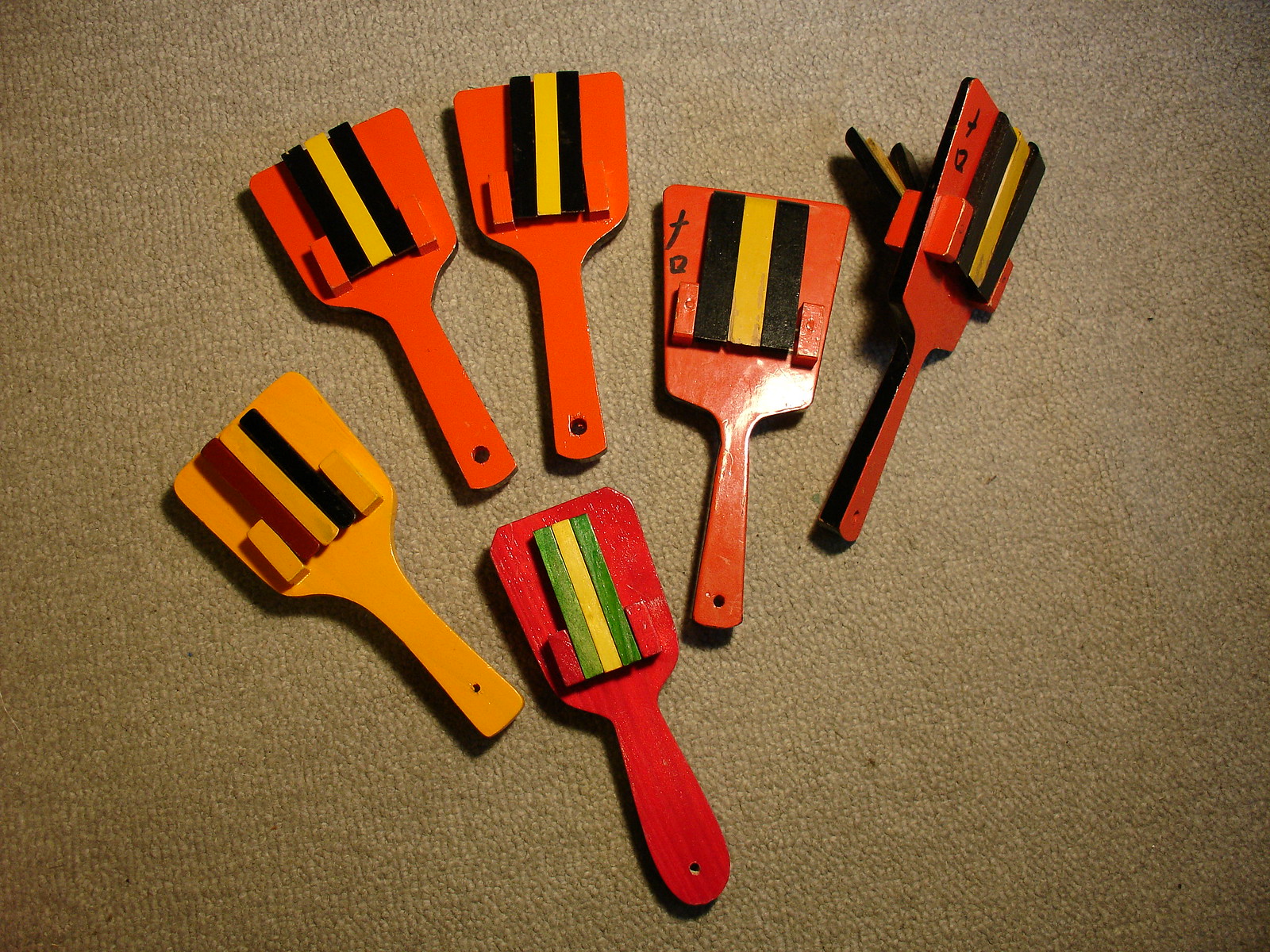The image depicts six wooden noisemakers laid out on a light brown, close-weave carpet. These objects are reminiscent of hairbrushes or paddles, lacking bristles, and each has a narrow handle with a hole at the bottom presumably for a string or handle attachment. The noisemakers vary slightly in shape, with some handles rounder than others, but all broaden out at the top, resembling the solid part of a fork without tines. They feature a series of raised blocks that create a tapping sound when shaken.

The predominant color of four of these noisemakers is orange, highlighted with black and yellow stripes. One of these orange noisemakers is positioned on its side, unlike the others, which lie face-up. Another noisemaker is red with a pattern of two small red stripes alongside longer green and yellow stripes. The final piece is yellow, adorned with brown, yellow, and black stripes. Some of the orange noisemakers additionally bear the marking "F.A." The noisemaker blocks are designed to move and create sound, suggesting a potential use as rhythm instruments or clappers.